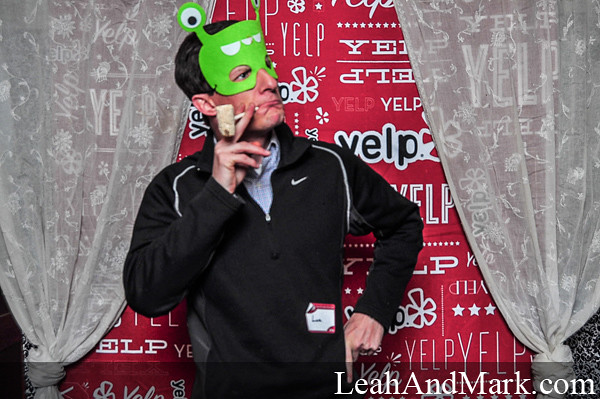The photograph captures a man standing indoors, seemingly at a festive event or party, against a busy red backdrop that prominently features the word “Yelp” and the Yelp logo repeated in various fonts. This eye-catching background is bordered by white, lacy curtains on both the left and right sides of the image, giving the impression of a photo booth setup. Positioned almost exactly at the center of the image, the man, who has short, dark hair and is Caucasian, wears a bright neon green paper mask designed to mimic an alien or monster, complete with a large, toothy smile and two eyeball stalks protruding from the top. 

He is dressed in a blue shirt under a long-sleeved black Nike pullover sweatshirt, with the Nike logo visible on his left breast. The man assumes a serious pose, with his head slightly turned to his left (our right) and his left arm placed akimbo on his hip. His right hand is slightly bent, holding a corncob pipe, which he has positioned in his mouth as a prop. The pipe is notably unlit, adding to the theatricality of his pose. 

The scene is detailed with the colors gray, red, white, light green, dark gray, and maroon. In the bottom right corner of the image, the website "LeahAndMark.com" is subtly included, with the L in Leah, A in And, and M in Mark capitalized.